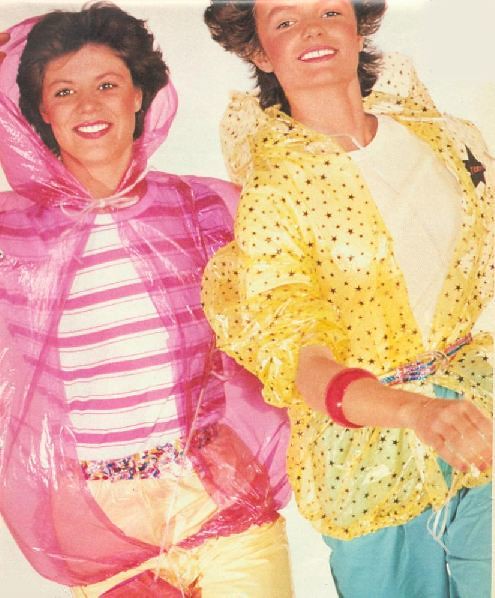In this detailed color photograph, likely from an early 1980s catalog, two adult Caucasian women with brown hair and blue eyes are posing side by side against a white backdrop, smiling directly at the camera. The woman on the left is wearing yellow pants, a floral belt, and a white and pink striped top. Over her outfit, she dons a see-through pink plastic rain jacket tied at the neck. The woman on the right is dressed in pale green pants and a white shirt with a pastel plaid belt. She complements her attire with a yellow transparent raincoat adorned with starry designs and a red wristband on her arm. The overall styling and vintage hairstyles suggest it's a fashion shoot showcasing retro raincoats, exuding an old-school charm reminiscent of 1980s catalogs.